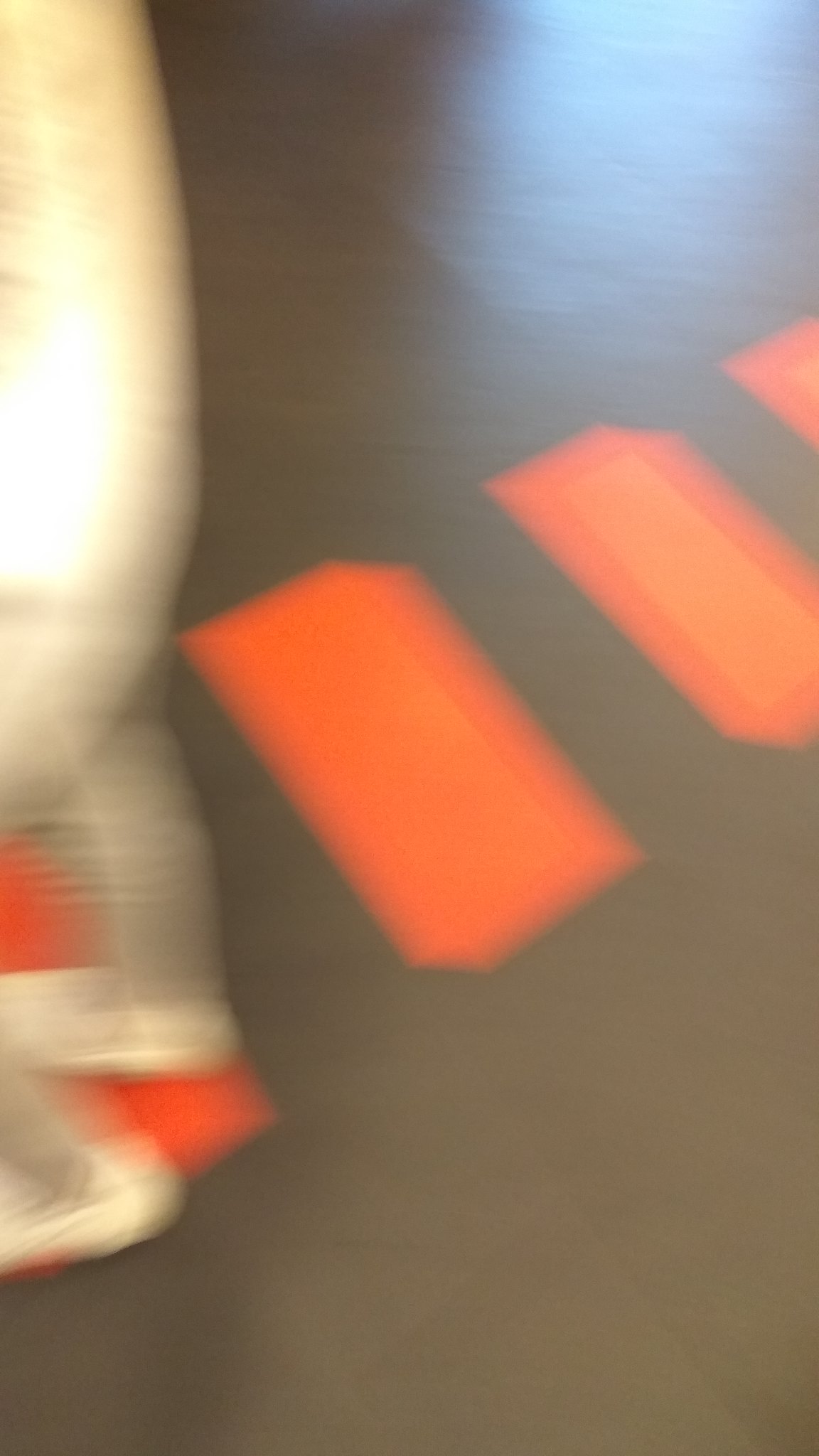The image depicts a shaky, blurry scene characterized by a series of four orange rectangles arranged on a dark gray floor, resembling a crosswalk or some kind of safety marking. Amidst the orange shapes, a pair of legs in light-colored pants and white or gray shoes are seen, giving the impression of someone walking across the path. The surroundings suggest a setting where caution or direction is indicated, possibly an indoor area like a gym. The overall background hue is a mix of gray and brown tones, with additional white and blue lights faintly visible, casting a glow from the edges of the image. The orange rectangles vary in intensity, creating a gradient from solid orange to orangey-yellow, adding a sense of depth despite the image's blur.